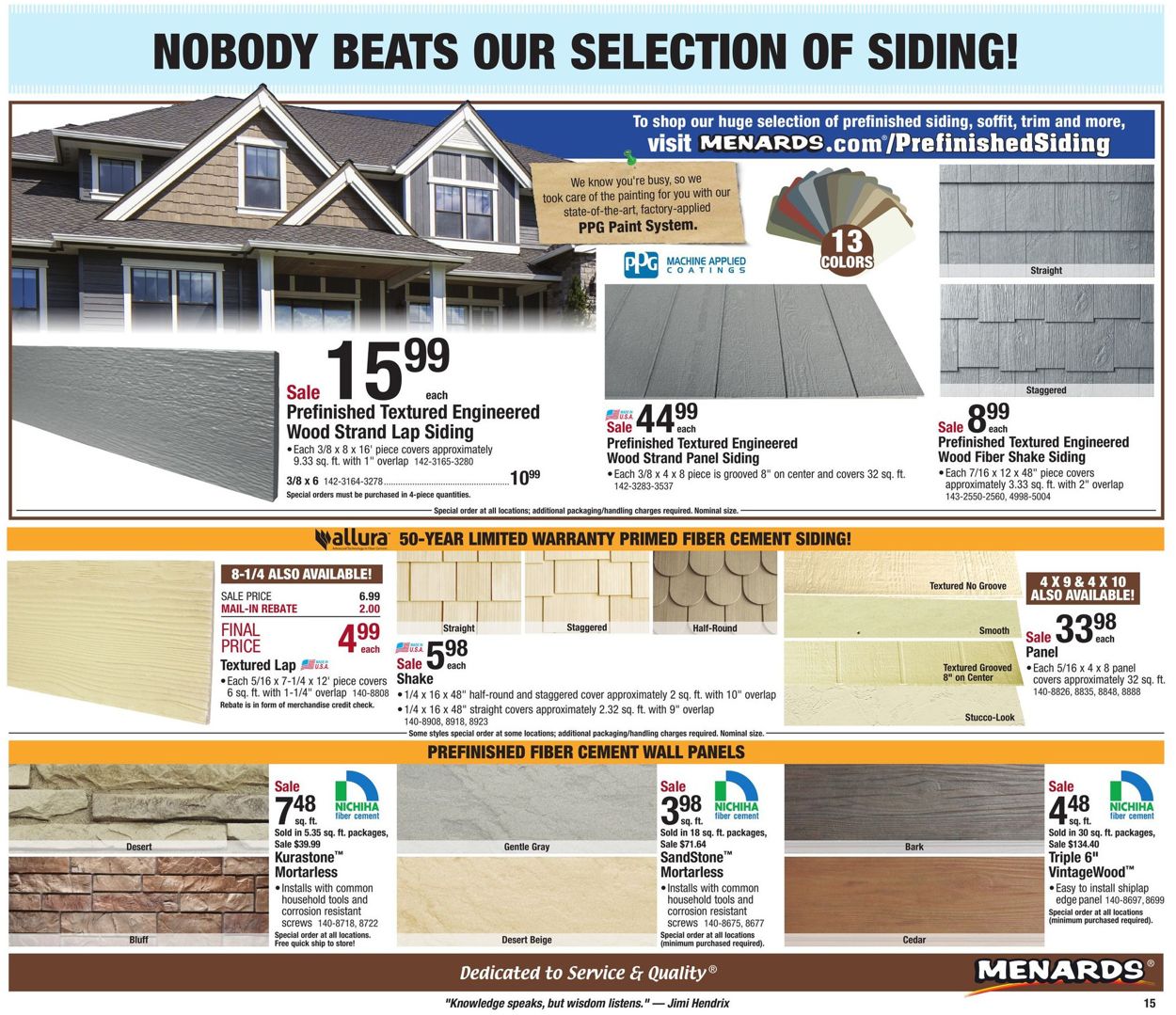This image is a screenshot that prominently features a promotional banner and detailed product information. At the top of the image, there is a light blue banner displaying bold black text in all capital letters that reads, "NOBODY BEATS OUR SELECTION OF SIDING." Below the banner, an illustration of a house is positioned on the left side, showcasing its front with brown siding. Underneath the house illustration, text indicates, "Sale $15.99 Prefinished Textured Engineered Wood Strand Lap Siding." To the left of this description, there is a close-up view of the siding to highlight its texture and appearance. On the right side of the image, another close-up view of siding is shown, labeled as "Prefinished Textured Engineered Wood Strand Panel Siding" in black text. The price for this product is listed beneath it in bold black text, reading "$44.99 each." In the upper right corner of the image, white text set against a dark blue background informs viewers to "To shop our huge selection of prefinished siding, soffit, trim and more, visit menards.com/prefinishedsiding."